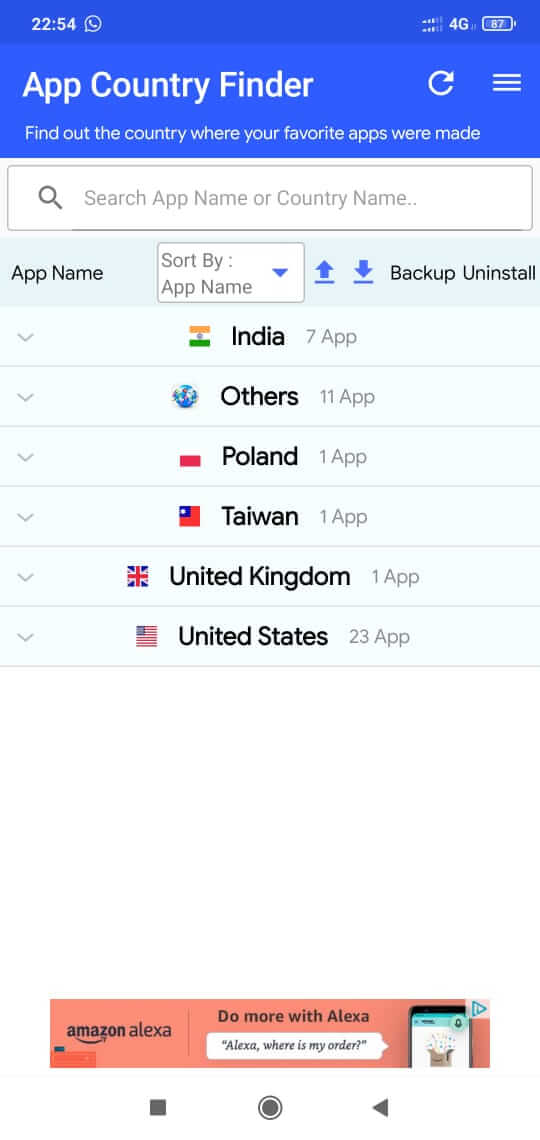This screenshot depicts the main interface of an application called "App Country Finder." At the top of the screen, a blue header bar spans across with the app's name, "App Country Finder," in white text centered. On the right side of this bar, there is a refresh button followed by a menu button represented by three horizontal lines.

Directly below the header, the app features a description: "Find out the country where your favorite apps were made," accompanied to the right by a white search bar that prompts users to "search app name or country name."

Beneath this section, there's a light blue area displaying the text "App Name" next to a white dropdown menu labeled "Sort by App Name." This section includes blue up and down arrows to facilitate sorting. Below these elements, users can see six dropdown boxes. Each box shows a country's flag, the country’s name, and the number of apps originating from there. The countries listed are India, Others, Poland, Taiwan, United Kingdom, and United States.

At the very bottom, a prominent orange banner advertises the capabilities of Amazon Alexa with the text, "Do more with Alexa." To the right side of the banner, there is an image of a phone, reinforcing the ad content.